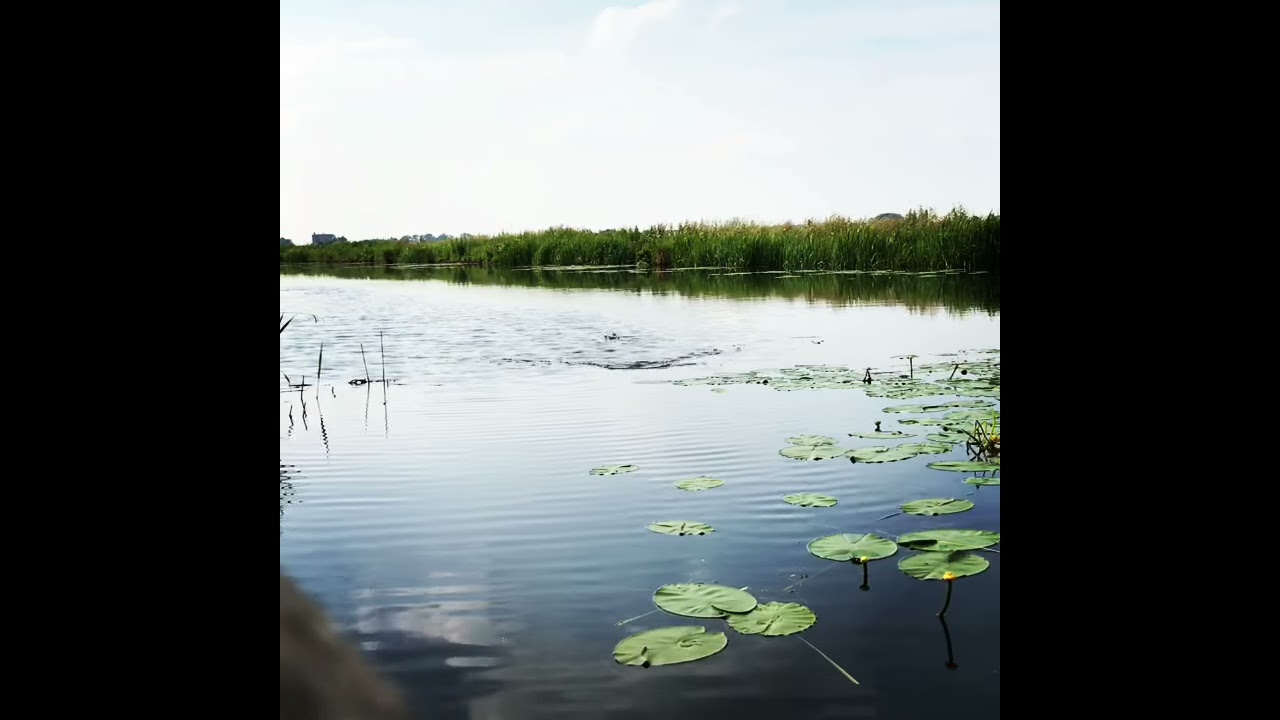This detailed photograph captures a serene and expansive lake or pond, stretching across the entire frame and flanked by black rectangles on both sides. The water is exceptionally clear and calm, with gentle ripples that reflect the pale sky, creating a mirror-like surface. Floating on the water are green lily pads, concentrated towards the bottom left of the image, while some grass and weeds emerge from the right-hand side. Surrounding the lake, lush greenery, including tall grasses and possibly mangroves, lines the banks. Trees and additional foliage can also be seen at the edges of the picture, casting their reflection onto the glassy surface of the water. The sky above is a very light blue, nearly white, filled with wispy clouds, suggesting either early morning or late evening light. In the center of the lake, there are small, barely visible figures that could be ducks, adding a touch of life to this tranquil scene. The overall composition is peaceful, highlighting the undisturbed nature of this idyllic setting.